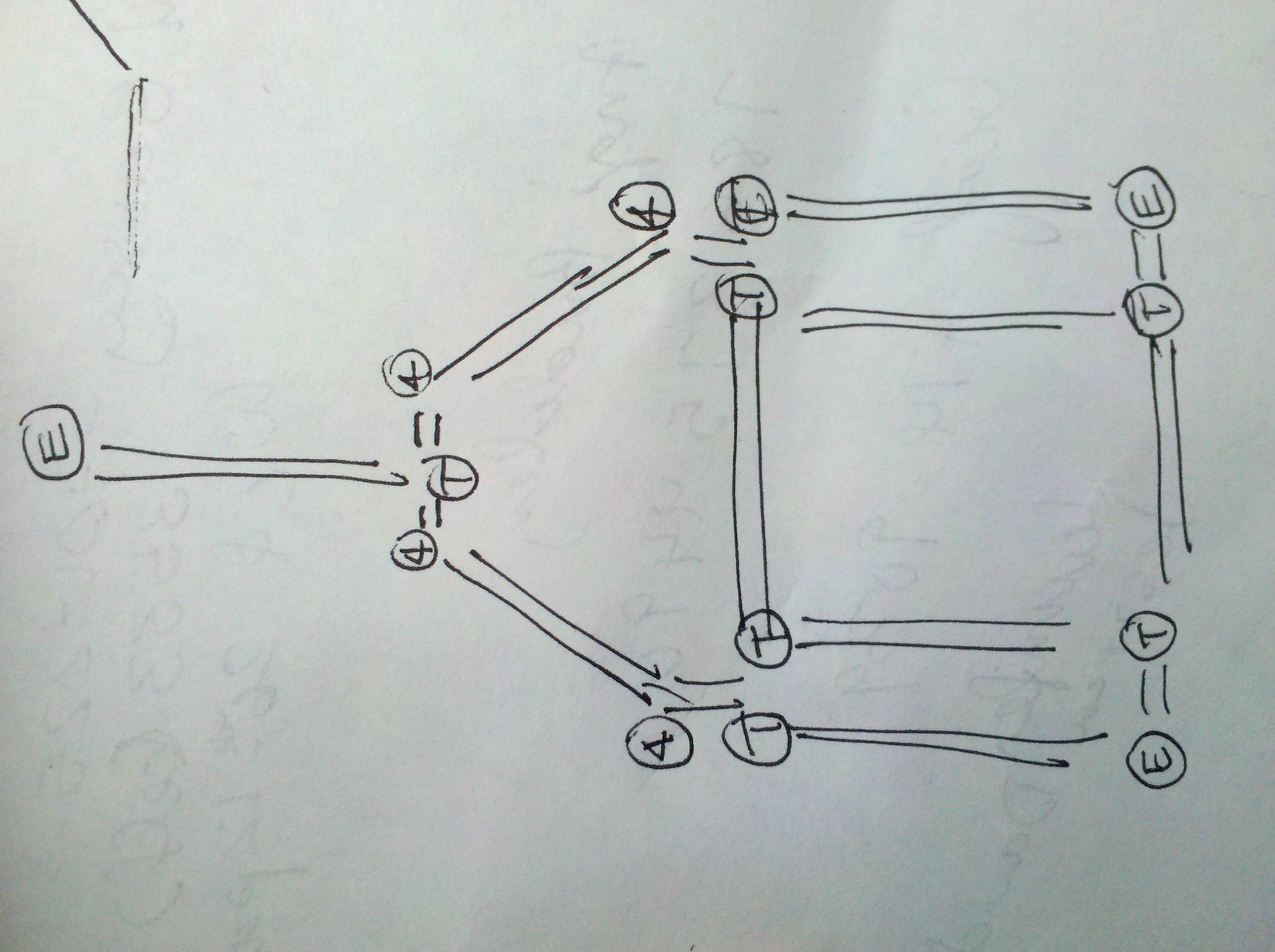The image depicts a meticulously drawn diagram on a white sheet of paper, illustrated using a black ink pen. The diagram features several round circles, each containing different numbers and letters. These circles are interconnected with double lines, forming a structure that resembles a sideways pyramid. Starting from the left side of the image, the first circled element is the letter "E," which connects to the letter "T" and the number "4," both also enclosed in circles. As the schematic extends rightwards, it branches out further into circles containing letters "A," "C," "T," and eventually culminates in a sequence of circled letters "E," "T," "T," and "E." Despite its precise construction, the purpose or meaning of this diagram remains unidentified.